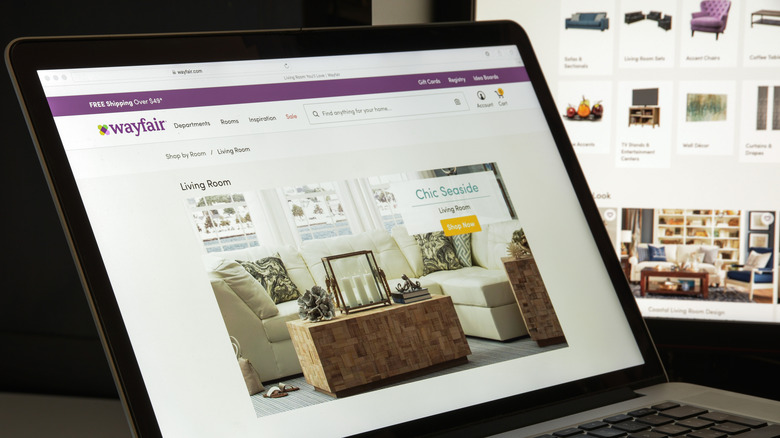In this image, we see an opened laptop displaying the Wayfair website. The screen showcases the Wayfair logo in the upper left-hand corner, written in distinctive purple letters. Above the logo, a purple banner stretches across the entire width of the screen, stating "Free shipping over $49." The main content on the screen features a section labeled "Chic Seaside Living Room," with "Chic Seaside" highlighted in green letters and "Living Room" in black just below it. An inviting yellow rectangle prompts users to "Shop Now" when hovered over with the mouse.

The highlighted item is a beautifully staged living room setup. Central to this setup is a pristine white couch, complemented by a brown wooden block coffee table positioned in front of it. The room is illuminated by natural daylight pouring in through the white-framed windows in the background, creating a cheerful and well-lit atmosphere. To the right of the couch, there is a matching end table that harmonizes with the design of the coffee table, completing this elegant, seaside-inspired living room scene.